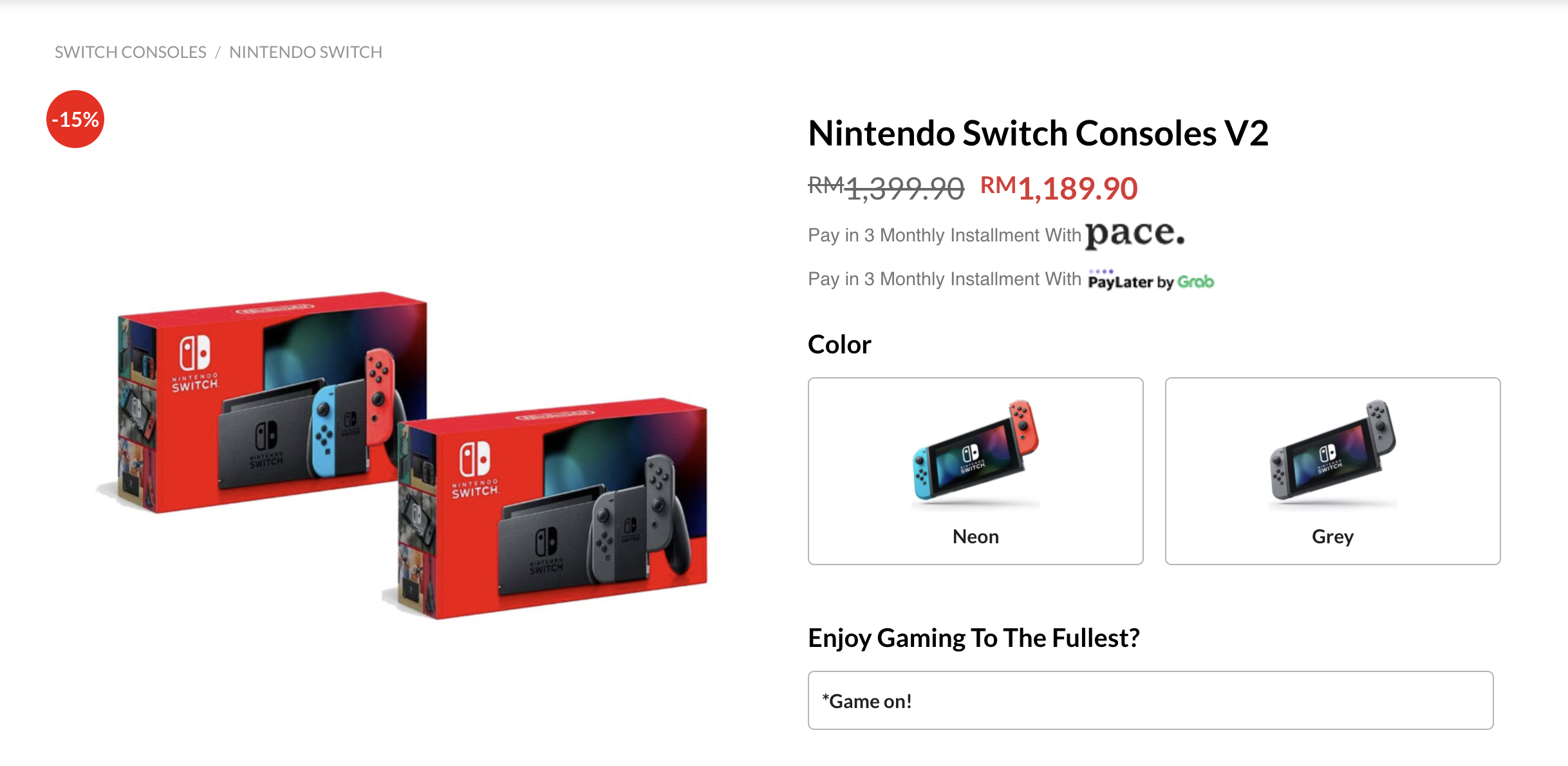The image showcases an advertisement set against a clean, white background. At the top of the image, in light gray, all-capital letters, the text reads "SWITCH CONSOLES / NINTENDO SWITCH." Just beneath this text, there is a circular badge displaying a discount of "15%" in white font.

Positioned below the badge are two boxed Nintendo Switch V2 consoles. The first box features a Nintendo Switch with neon blue and neon red Joy-Cons, while the second box features a Nintendo Switch with gray Joy-Cons. Both boxes are labeled "Nintendo Switch consoles version 2."

The initial price of the consoles is marked as $1,399.90, but it is reduced to $1,189.90. The advertisement also highlights payment options, specifying that you can pay in three monthly installments either with Pace or via Pay It Later by Grab.